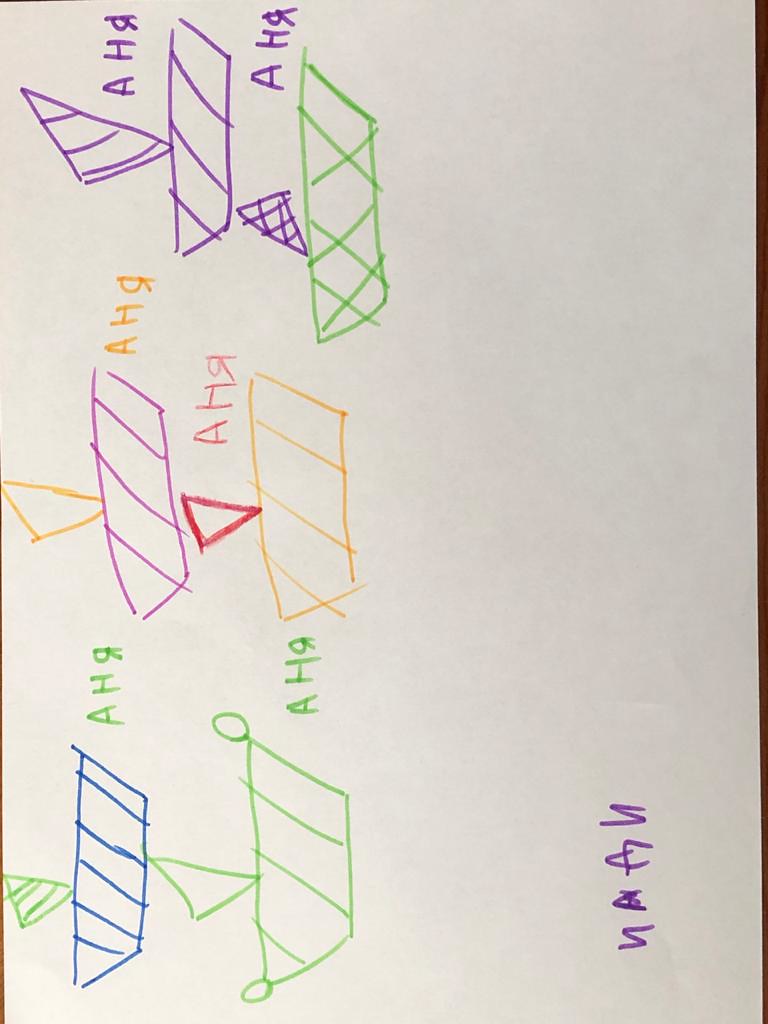The image captures a white rectangular piece of paper positioned vertically on a brown table. The paper is filled with repetitive doodles, each featuring an angled rectangle balanced atop a triangle. The sketches are meticulously organized into three horizontal rows of two pairs each. 

- The top row features doodles with the left being predominantly purple and the right predominantly green.
- The middle row has a mix of purple and orange on the left doodle, while the right one combines orange and red.
- The bottom row displays a left doodle with blue and green shades, while the right one is entirely green. 

All the doodles bear identical labels that include the capital letters A, H, and a backward R, presented in varying hues of purple, orange, red, and green. In some images, there are small circles, particularly noticeable in the bottom right doodle.

A few unintelligible letters are scribbled at the bottom right corner of the paper, resembling someone testing the ink of their pen. It's noteworthy that none of the doodles are colored in but are instead filled with simple line drawings. Despite the vertical orientation of the paper, the arrangement of the doodles suggests that the image might have been more fitting taken horizontally.